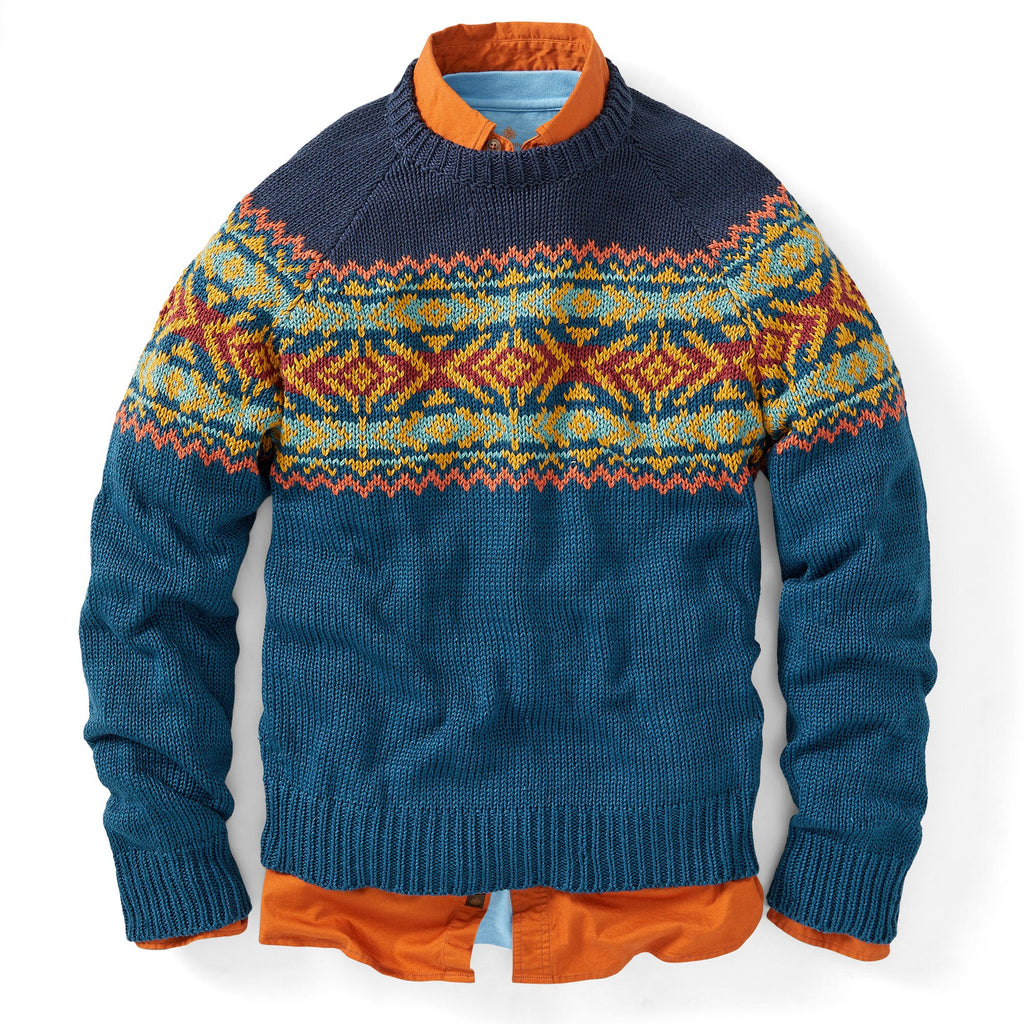This is a detailed square-format color photograph depicting a set of clothes arranged as if worn, yet floating against a white background. The central piece is a long-sleeved sweater, predominantly medium blue with a lighter blue lower section. The sweater features an intricate horizontal stitched pattern across the chest and upper arms. This pattern starts with a zigzag stitch in pinkish-orange on the top and bottom edges, followed by bands detailed with red, blue, and gold. The central part of this design showcases yellow diamond shapes with smaller red diamonds within, set against a blue background. This decorative band gives the appearance of traditional motifs often seen in textile arts. Underneath, an orange button-up collared shirt is layered over a white t-shirt, providing a contrasting pop of color. The photograph adopts a style of photographic representationalism, capturing the realism typically employed in fashion photography, as it presents the garments in a clean and appealing manner suitable for a retail website.